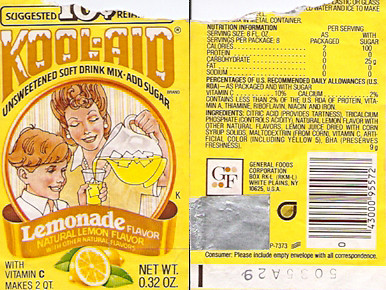The image showcases a retro-styled, yellow Kool-Aid package, designed to look vintage. The package is torn across the top and spread open, revealing both the front and back. Prominent on the front is the text "Kool-Aid" in an orange color with a snowy white outline, suggesting a frozen theme. The package originally retailed for 10 cents, although the price is partially torn away. Below the Kool-Aid logo, it states, "unsweetened soft drink mix, add sugar," in black print. A circular illustration depicts a smiling Caucasian woman pouring lemonade from a clear pitcher with ice into a glass held by a boy. Both of their eyes are closed. Beneath this image, the text reads "lemonade flavor, natural lemon flavor with other natural flavors," alongside a halved yellow lemon graphic. 

The package indicates it contains vitamin C and makes two quarts of the drink, with a net weight of 0.32 ounces. On the lower left of the front, it emphasizes the presence of vitamin C, while the lower right notes the net weight. The back of the package features nutritional information, a General Foods (GF) logo, and their address. There's a barcode and a batch identification code "5035A29," which suggests it is designed to appear older than it is due to the presence of modern barcode technology.